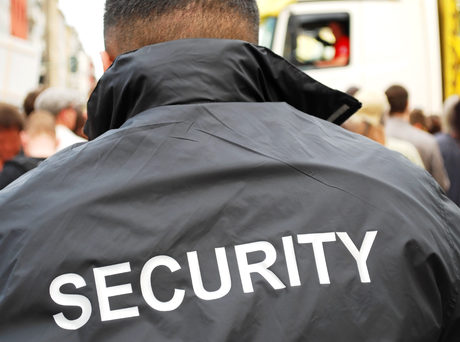In this close-up photograph, we see the back of a security guard, distinguishable by his black nylon jacket with a slight shine. Prominently centered on the back of the jacket, in bold white letters, is the word "SECURITY." The jacket features a thick collar that is partially standing up at the back of the guard's head, which is shaved on the bottom half with slightly longer, very short hair on top. The background is out of focus, illustrating a bustling crowd of people and various elements like a semi-truck with a cab in the left corner. Through the truck's window, a man in a red shirt is visible, though blurry. Partially visible around the security guard are multiple individuals, including a person with dark brown hair in a gray shirt, another with salt and pepper hair in a light blue t-shirt, and another figure with an olive complexion and white shirt. The image is taken during a gray day, as indicated by the overcast sky.